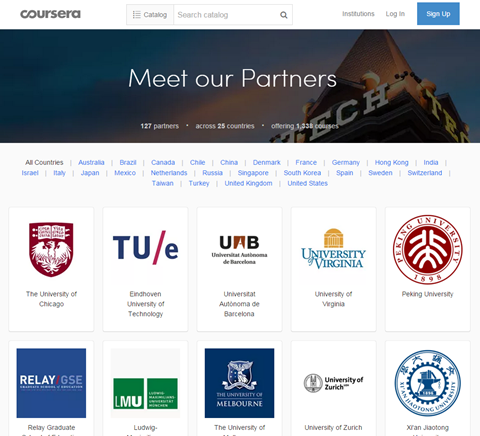This is a cropped screenshot of the "Meet Our Partners" page on the Coursera app. At the top left, the familiar Coursera logo is prominently displayed. To the right of the logo, there are two navigation elements: a category selection, followed by a search bar. On the far right, options for "Instructions," "Log In," and "Sign Up" are available, with the "Sign Up" button highlighted in a blue box.

Beneath the top navigation, a large rectangular banner is featured, displaying the text "Meet Our Partners." Below this, three company names are listed as bullet points.

The bottom section of the page is dedicated to content categories and course thumbnails. At the very top of this section, an "All Categories" button is visible, followed by several horizontal lines of category selections. Beneath the categories, there are ten thumbnails arranged in two rows of five. Each thumbnail features an icon at the top, with the associated school name displayed below it. The thumbnails are not numbered or ranked.